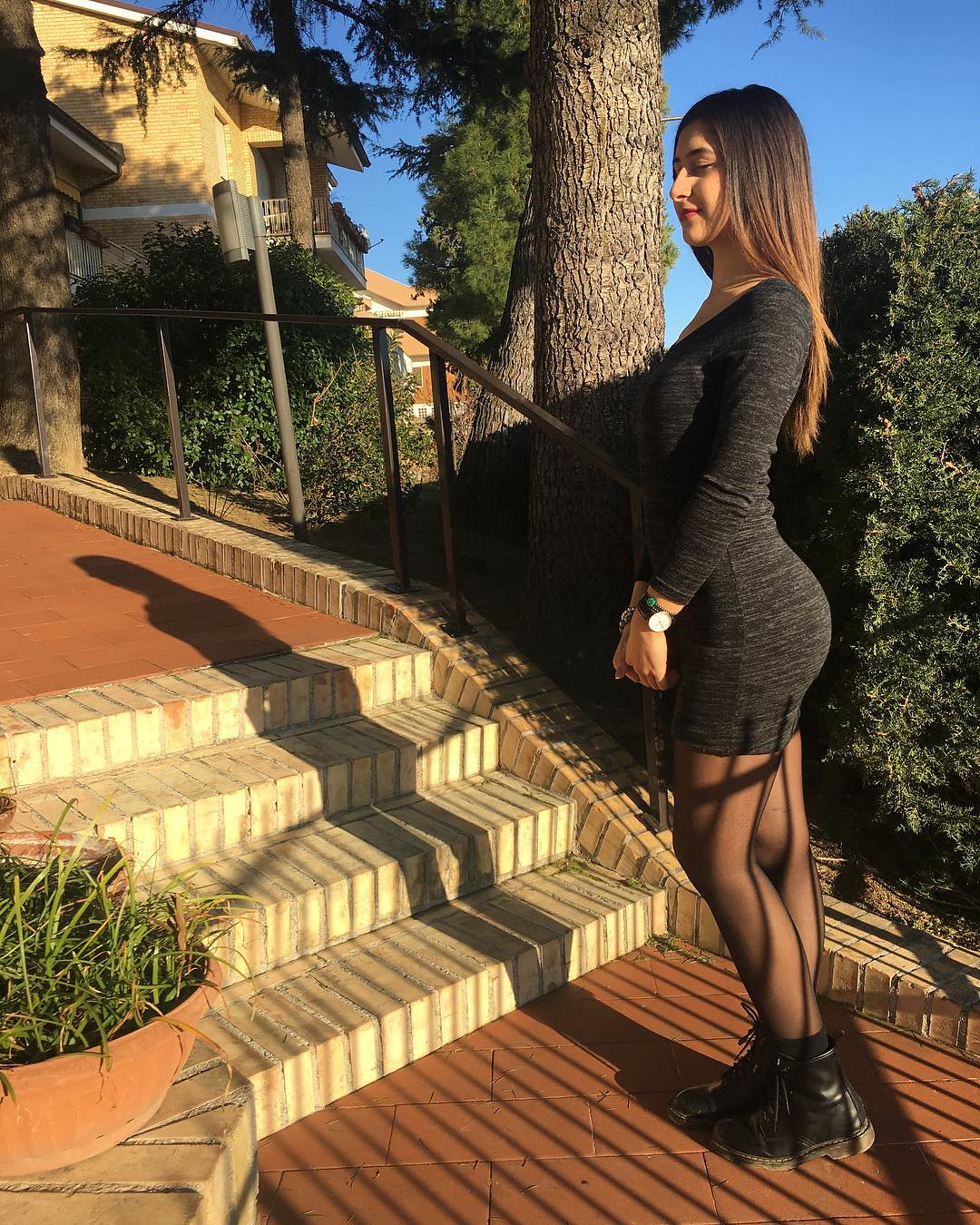A lady with long brown hair, featuring an ombre effect that transitions from dark at the top to lighter at the bottom, stands outdoors in front of a set of beige brick steps on the left side of the image. The steps ascend to a maroon brick area. She occupies the right side of the image from top to bottom, facing the steps with a slight smile, her eyes closed, and her hands held demurely in front of her. She is wearing a form-fitting black dress with gray striations, gray stockings, and black boots. A watch adorns one of her wrists. To the lower left, there is a clay pot with green grass on a stone wall. The background includes bushes, trees, and a yellow brick house with red material accents. Additionally, a patch of clear blue sky is visible in the upper part of the image.